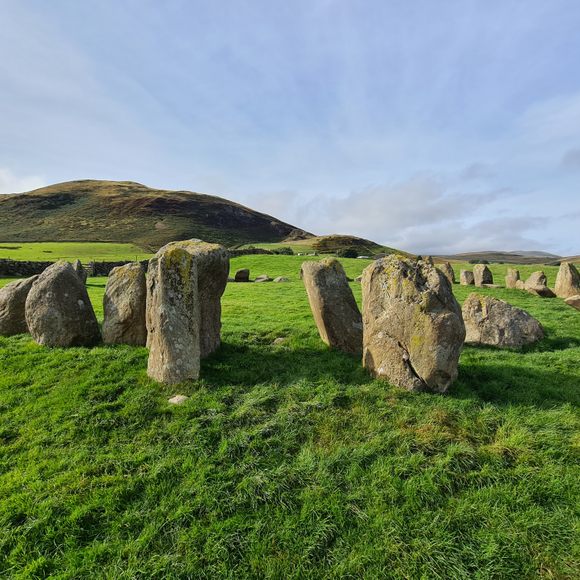The photograph is a realistic, square-shaped, outdoor scene depicting a sunny day with a light blue sky dotted with thin white clouds. Dominating the middle and bottom sections of the image is a lush, green grassy field transitioning into a gently sloping hillside in the background. Central to the photograph is a purposeful arrangement of large stones, reminiscent of a smaller Stonehenge. These stones, each roughly the size of a large, thick suitcase—about two to three feet high and wide, and around a foot thick—are weathered and covered in patches of moss and algae, giving them an aged and natural appearance. Additional stones can be seen lying on the ground and in a line across the middle ground, enhancing the deliberate arrangement. In the background, the greenery gives way to hills and possibly mountains, where the vibrancy of the grass diminishes slightly. The scene is well lit, suggesting it's relatively sunny, and the overall ambiance is peaceful and picturesque with natural elements harmoniously arranged.